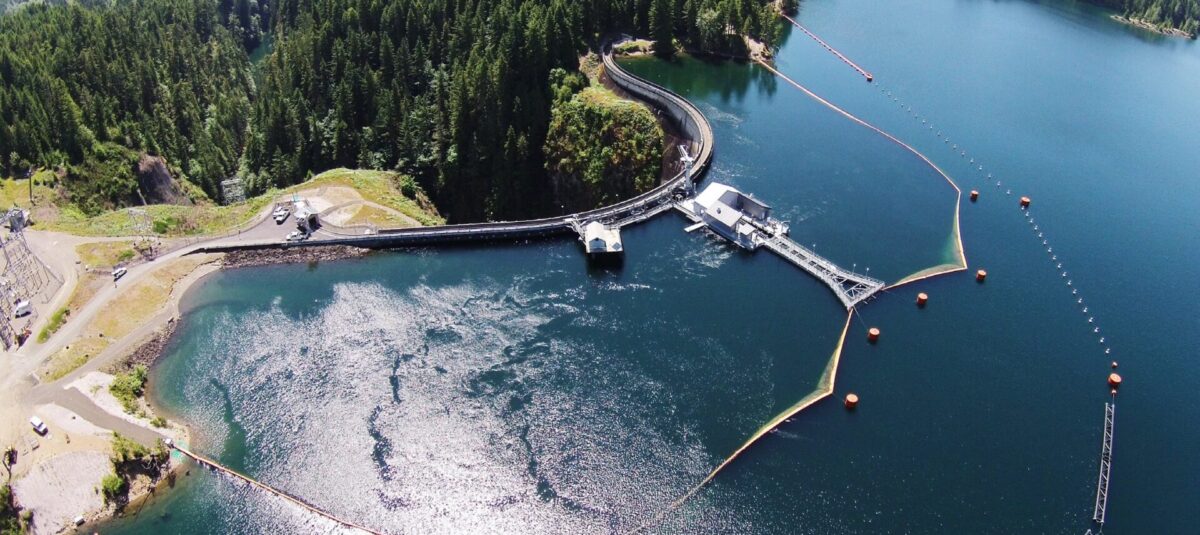An aerial, slightly angled photograph captures a unique body of water, possibly a lake, that appears almost as if it's floating. A dam or some sort of man-made structure borders part of the water, creating an illusion that the lake is perched on the edge of a drop-off, leading straight to a dense forest where only the tops of the trees are visible. At the upper part of the image, the landscape transitions sharply from water to forest, suggesting the water might be disappearing off a cliff or hill. The water itself is sectioned off with what appears to be ropes or nets, creating distinct areas within the lake. A pair of white boats, with one being noticeably larger and possibly pulling something, are engaged in some activity—possibly working with a net that is mostly submerged and looks almost solid, like a tarp. The scene resembles a construction site, reinforced by the presence of a small building and various trucks parked in the dirt along the edge of the water. Buoys and other man-made items also dot the area, adding to the industrial feel of the landscape.